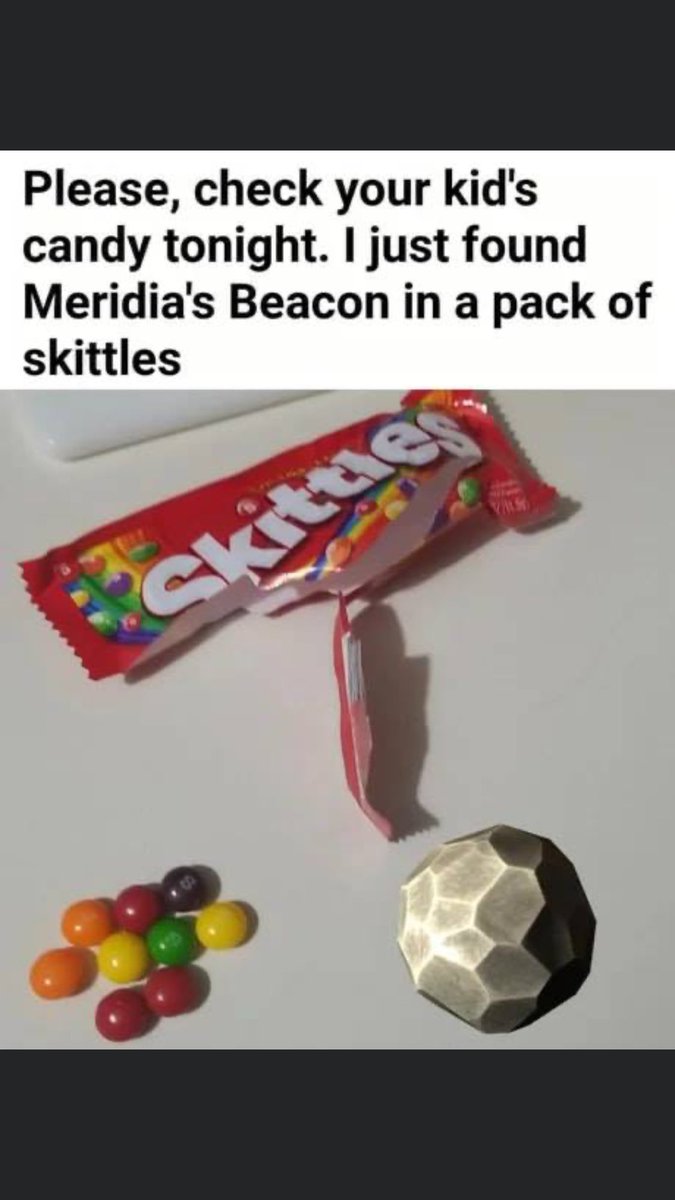The image depicts an open bag of Skittles with its colorful contents spilled onto a hard, white surface, likely a table. The Skittles are red, orange, yellow, green, purple, and brown. Amidst the scattered Skittles is a peculiar hexagonal ball that appears superimposed, likely added for a humorous effect. Above the scene is black text on a white background that reads, "Please check your kid's candy tonight. I just found Meridia's Beacon in a pack of Skittles." This statement seems to reference an inside joke or cultural meme, possibly unfamiliar to some viewers. The Skittles package is standard, emphasizing the contrast with the unusual hexagonal object among the candies.